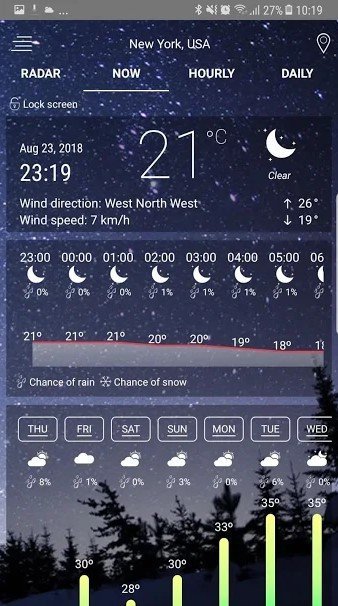Screenshot of a Weather Application on an Android Smartphone

This image captures a screenshot from an Android smartphone displaying a weather application for New York. The smartphone interface, located at the top right, includes various Android status icons: the Bluetooth emblem, a muted sound symbol (indicating the phone is on vibrate mode), an alarm clock icon (indicating an alarm is set), a Wi-Fi logo (showing an active connection), and full cell phone data signal. The battery life stands at 27%, denoted by a battery icon, and the current time is 10:19 PM (2319 in 24-hour format), inferred from the nighttime theme.

The weather app reveals that on August 23rd, 2018, the current weather in New York is clear with a temperature of 21 degrees Celsius. The night sky is illustrated with a moon icon. Moreover, the application provides comprehensive meteorological details such as wind direction, phases of the moon (waxing/waning, full moon, or half moon), and a weekly weather forecast spanning from Thursday through Wednesday.